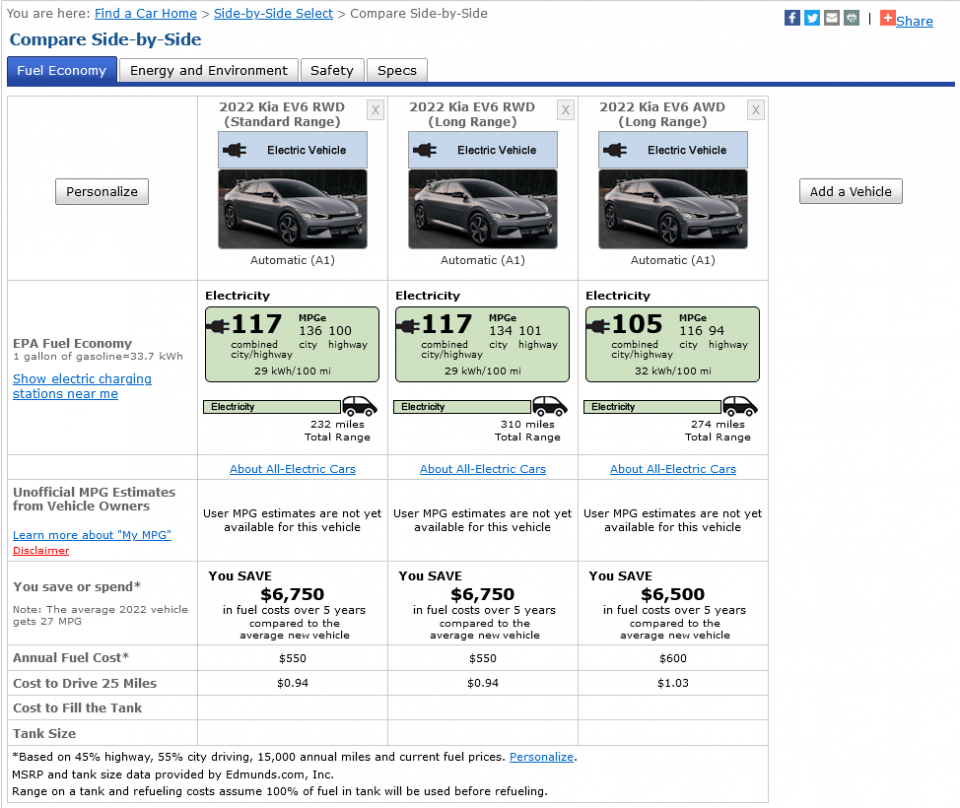In the image, the top section displays the text "You are here. Find a car: Home >> Side-by-Side." On the right side, there is a blue button that says "Compare Side-by-Side." Below this are several grey tabs labeled "Fuel Economy," "Energy and Environment," "Safety," and "Specs." The "Fuel Economy" tab is highlighted in blue, indicating the current view.

The image shows a comparison of three cars, all of which are the same model: the 2022 Kia EV6 Rear-Wheel-Drive. They are all automatic electric vehicles and are depicted in a slightly black color. The first car is the Standard Range model, the second is the Long Range model, and the last is the Long Range All-Wheel-Drive model.

For each car, the electricity output is displayed in green. The Standard Range and Long Range models both have an electricity output of 117 MPGe, while the All-Wheel-Drive model has 105 MPGe. 

Additionally, the image provides details on fuel cost savings over five years. The Standard Range and Long Range models both indicate a fuel cost saving of $6,750, while the Long Range All-Wheel-Drive saves $6,500 over five years. The total range in miles for the Standard Range model is 232 miles, for the Long Range model is 310 miles, and for the Long Range All-Wheel-Drive model is 274 miles.

The background of the image is white, and in the top right corner, there is a button labeled "Add VIP," allowing users to add another vehicle for comparison. The electricity output or MPGe values are highlighted in green for clarity.